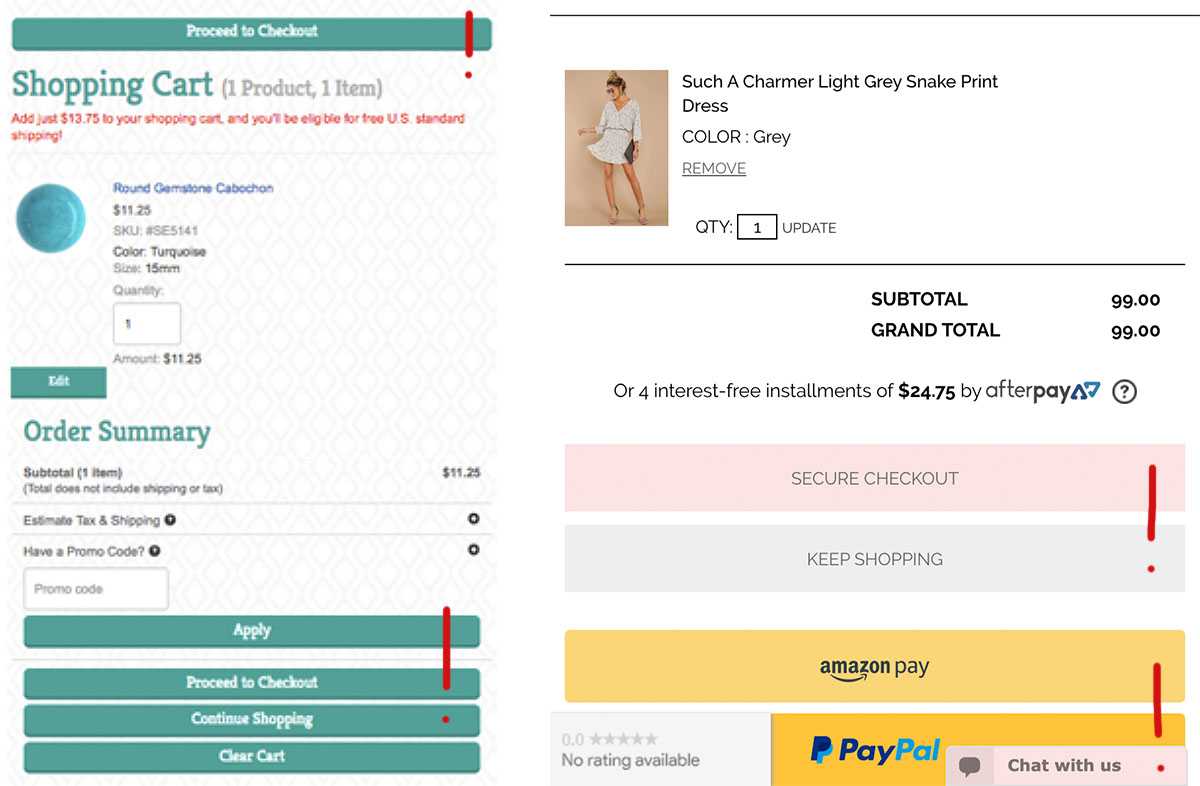This image displays a dual screenshot of a website checkout process, providing an in-depth view of a shopper’s cart and various payment methods. 

**Left Section:**
- A teal button at the top labeled "Proceed to Checkout," with "Shopping Cart" below it, indicating there is one item in the cart.
- A red notification states, "Add $13.75 to your shopping cart to be eligible for free US standard shipping."
- The item summary features a small, blue, marbled circle representing the product, accompanied by the title "Round Gemstone Cabochon."
  - Price: $11.25
  - Color: Turquoise
  - Size: 15mm
  - Quantity: 1
  - Total: $11.25
- Below this is a green "Edit" button.
- An order summary provides details on estimated tax, shipping options, and promo code entry fields.
- Additional action buttons include "Apply," "Proceed to Checkout," "Continue Shopping," and "Clear Cart," all in teal color.
- A red exclamation point suggesting important information or an alert.

**Right Section:**
- The upper part directly shows an image of a woman in a dress with the item details on the right:
  - Item: "Such a Charmer Light Grey Snake Print Dress"
  - Color: Grey
  - An option to remove the item from the cart
  - Quantity: 1
- The pricing summary shows:
  - Subtotal: $99
  - Grand Total: $99
  - Alternatively, "4 installments of $24.75 by Afterpay."
- Below the total price, there are two options: a pink "Secure Checkout" button and a grey "Keep Shopping" button.
- Another red exclamation point is visible on the right, catching attention for some important notice.
- Different payment options are displayed, including:
  - Amazon Pay (yellow button)
  - PayPal (yellow button)
- Zero grey stars, indicating no ratings are available.
- A pink "Chat with Us" button for customer support.
- Yet another red exclamation point on the far right, indicating possibly critical information or instructions.

The well-detailed presentation ensures that the shopper has clarity on the items, payment methods, promotional details, and any actions needed for finalizing the purchase.